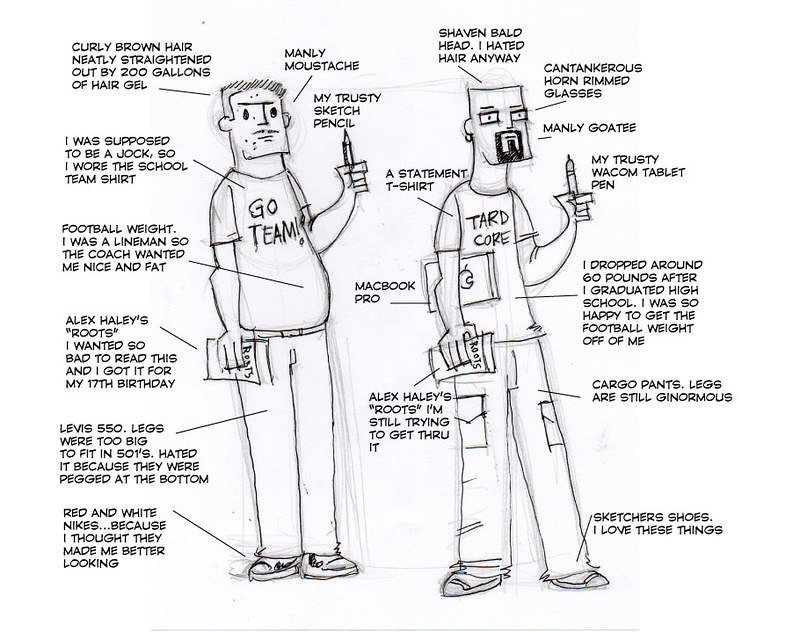This black-and-white sketch depicts two men, each surrounded by detailed annotations about their appearance and accessories. The man on the left, with curly brown hair heavily styled with hair gel, sports a manly mustache and wears a school team shirt representing his former role as a football lineman. His annotations reveal a desire to read "Alex Haley's Roots," gifted to him on his 17th birthday, and his struggle with wearing Levi's 501 jeans. He completes his look with red and white Nikes. 

On the right, the second man features a shaved bald head, cantankerous horn-rimmed glasses, and a manly goatee. He holds a Wacom tablet pen and a MacBook Pro, indicative of his current tech-savvy lifestyle. This man also carries an enduring interest in "Alex Haley's Roots," though he's still reading it. He proudly notes shedding 60 pounds post-high school and now wears cargo pants with Skechers shoes. The juxtaposition of their former and current selves, described with precision, offers a commentary on personal growth and change over time.